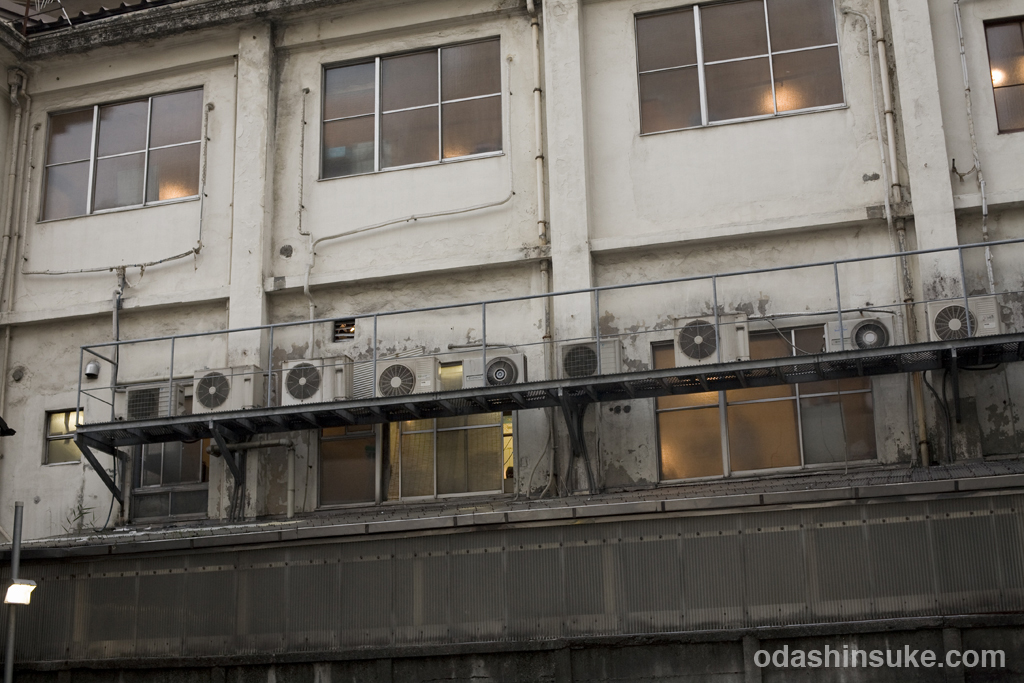The image depicts a fairly old, sturdy building, predominantly painted white, with patches of brown and signs of dirt and grime along its sides. The structure features multiple floors, though only part of it is visible. The visible upper windows, each divided into six panes with the possibility of being slideable, have lights shining through them, emitting a warm orange glow from ceiling fixtures inside. The lower part of the building includes additional windows bordered by metal railings, with air conditioning units mounted below some of the windows. Pipes run vertically and horizontally along the building’s exterior, and a bit of greenery can be seen near the base. There is a light fixture projecting downwards onto an unseen sidewalk or street. The building also has opaque windows on what looks like a walkway and some parts exhibit brownish and white grading, hinting at the practical nature of the building, possibly a warehouse. The bottom of the image contains text reading "odashinkingsu.com."